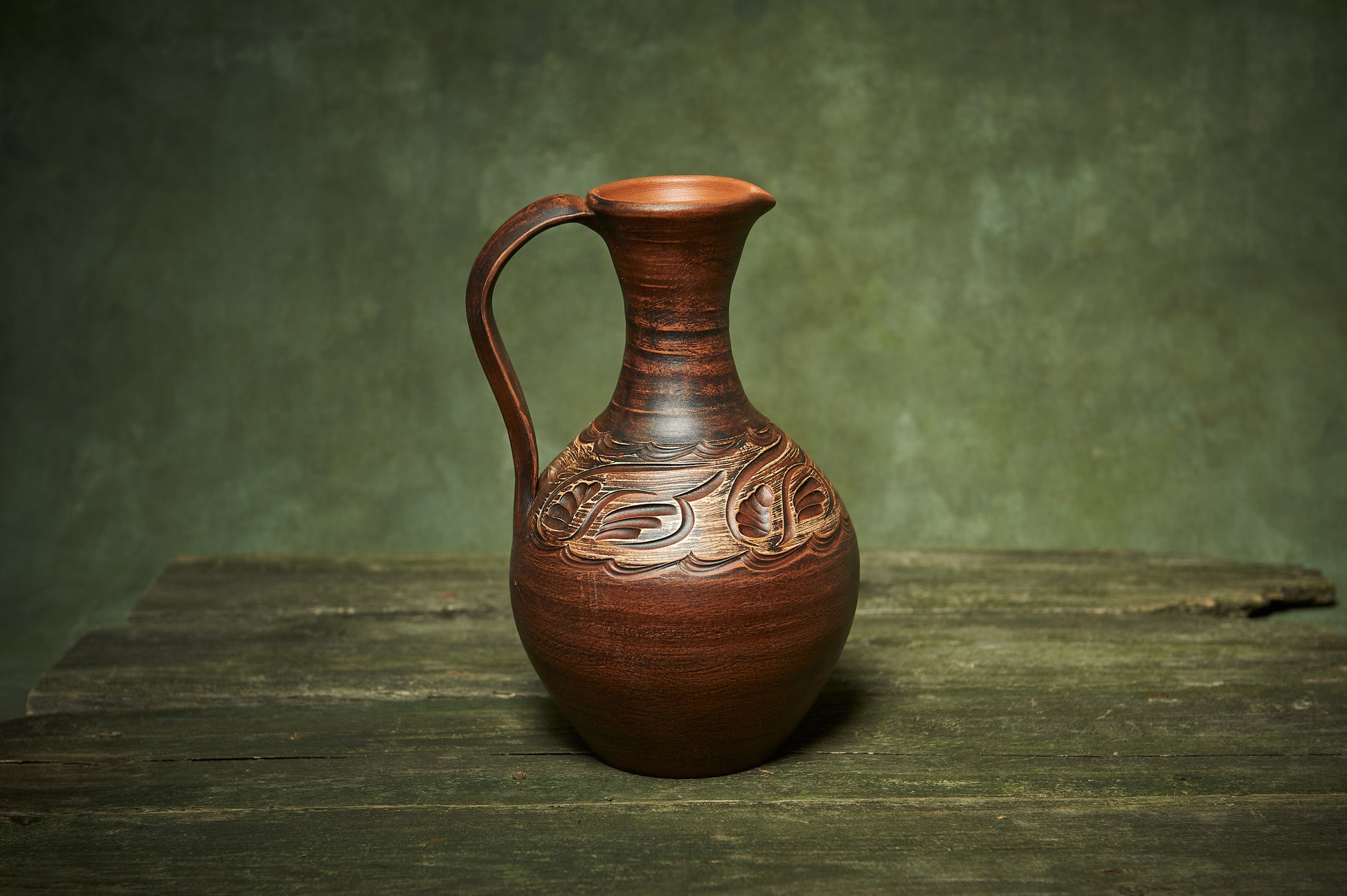This photorealistic image features a wooden vase with a highly polished dark wood grain. The vase showcases a decorative, etched pattern reminiscent of waves or water, and has a distinctive shape: starting wide at the base, it widens further in the middle, then narrows at the neck before flaring out slightly at the spout. A thin handle extends from the top of the vase down to the wider base. The vase rests on an old, unfinished wooden table, and the background features a green, brushed texture. The combination of lighting and composition suggests a carefully curated photograph, perhaps intended for an online listing.